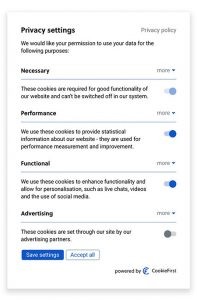The image displays a computer screen showcasing the privacy settings interface. The heading indicates a request for user permissions to use data for various purposes. Each category, including "Necessary," "Performance," "Functional," and "Advertising," has a detailed description and a "More" option for additional information.

- **Necessary:** This category highlights that certain cookies are essential for the website's functionality and cannot be turned off. These cookies ensure the site operates correctly.
  
- **Performance:** These cookies gather statistical information to measure and improve the site's performance. The setting is enabled by default, but users have the option to disable it.
  
- **Functional:** Cookies in this category enhance website functionality and personalization features such as live chat, videos, and social media integration. This setting is also enabled by default but can be turned off by the user.
  
- **Advertising:** Set by advertising partners, these cookies manage advertising content. This setting is currently disabled.

At the bottom left-hand side of the screen, there are two buttons: "Save Settings," which saves any changes made, and "Accept All," which enables all settings.